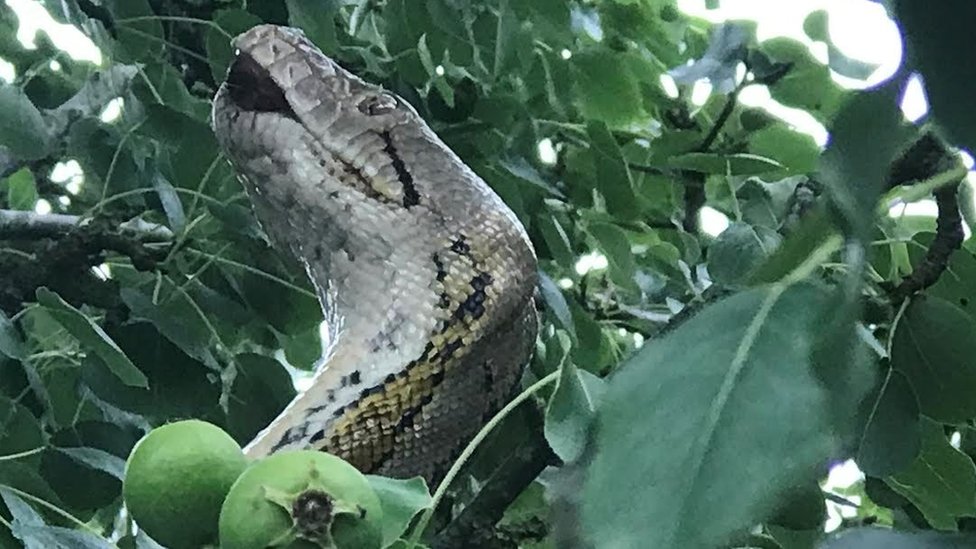In this horizontally oriented, color photograph of an outdoor scene, the prominent feature is the head and neck of a large snake, which are centered in the image. The snake's head, sporting a silver-gray color with some greenish tints, is pointed slightly upward and to the left. The snake's body, adorned with black stripes and gold accents, along with silvery eyes possessing tiny black pupils, extends and disappears behind some green, round fruits at the base of the photo towards the left. Surrounding the snake are numerous lush tree branches adorned with heart-shaped, pointed green leaves that filter the light. A bright white sky is visible through the foliage, most prominently in spots at the upper right and upper left corners. Additional spots of light shine through the leaves, gently illuminating the scene.